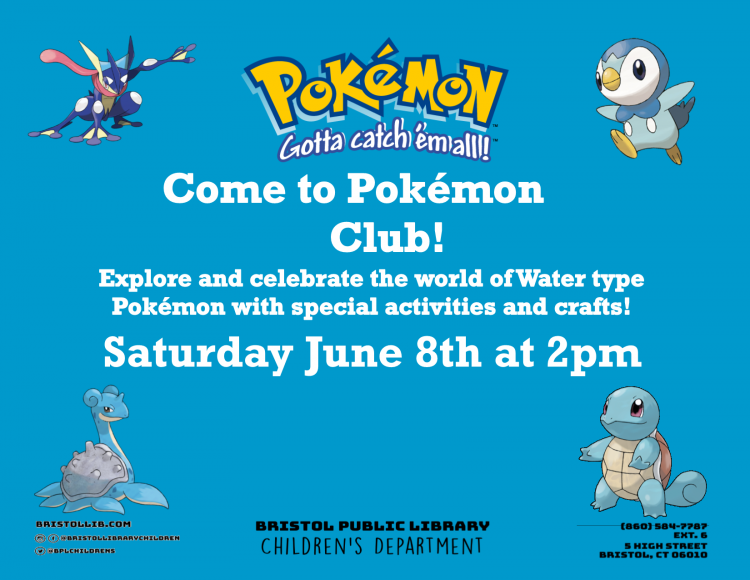This is a detailed description of an advertisement for the Bristol Public Library Children's Department. The ad features a light sky blue background with a rectangular shape. Each corner of the rectangle showcases an image of a different Pokémon character: a dragon-like Pokémon in the top left, a bird or penguin Pokémon in the top right, a turtle-like Pokémon in the bottom right, and a sea creature, possibly a seal, in the bottom left corner.

At the center of the advertisement, in bright yellow font with a dark blue outline and light blue shadow, is the word "Pokémon," curved elegantly. Directly below it, in white font, is the phrase "Got to catch them all!" with an exclamation point for emphasis. Beneath this, the text transitions to a straight font and reads "Come to Pokémon Club!" accompanied by another exclamation point. The ad concludes with the event details: "Saturday, June 8th at 2 p.m."